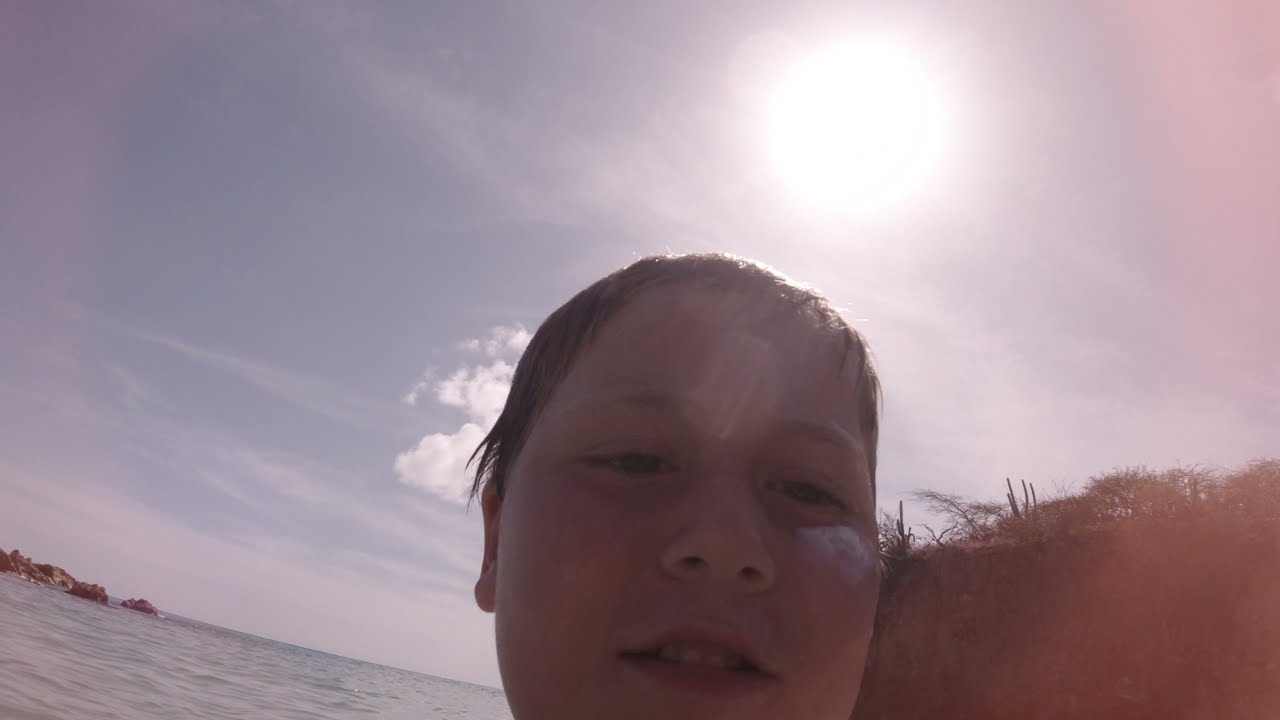A close-up photo captures a young Caucasian boy, around nine or ten years old, with short, wet brown hair, and narrow blue eyes. His face fills most of the frame, with only a bit of his ear visible on the left side, and the bottom lip and chin cut off. His mouth is slightly open, revealing the top row of his teeth, and he appears to be looking downward at the camera, which suggests he is taking a selfie. The background shows a mix of natural elements: directly behind him is a body of rippling water with some rocks emerging at the lower left corner, indicating a lake or an ocean setting. The sky, filled with clouds, has patches of blue and some white clouds that partially obscure the sun, which casts a warm, reddish glow, especially on the right side of the image. To the right of the boy, a landscape of vegetation, including sticks and brush, can be seen on a small hill. The overall scene depicts a bright, warm day with the boy enjoying his time outdoors, possibly having just come out of the water.